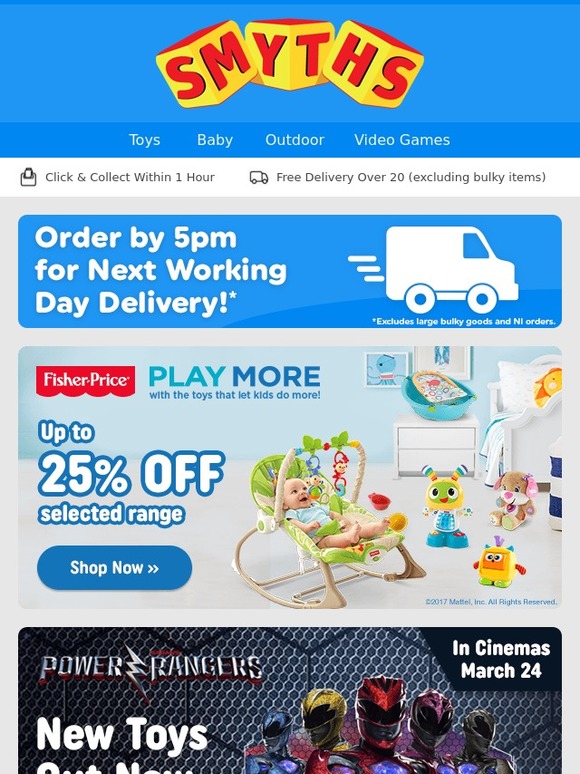This screenshot from a smartphone displays an advertisement for a toy store under the header "Smurfs MSYTHS," with the letters "SM" and "YT" highlighted in red on yellow building blocks. Below the header, there's a navigation bar listing categories: "Toys," "Baby," "Adorable," and "Video Games," alongside offers such as "Click and collect within one hour" and "Free delivery on orders over £20, excluding bulky items."

Further down, a blue box indicates: "Order by 5pm for next working day delivery from Nick's store." This is accompanied by an icon of a speeding delivery truck. A small note below specifies that the store excludes large bulky goods and Northern Ireland (N.I.) orders.

Central to the advertisement is the Fisher Brush logo with the tagline "Play more with the toys that kids love." It boasts a discount offering "Up to 25% off selected range," next to a prominent blue "Shop Now" button. To the right, an image features a baby in a green cradle surrounded by toys. Additional imagery includes toys on a dresser, on the floor, and on a bed, with pictures on the wall above them.

The bottom section against a black background promotes the "Power Rangers" movie, hitting cinemas on March 24th, accompanied by new toys and images of the five Power Rangers.